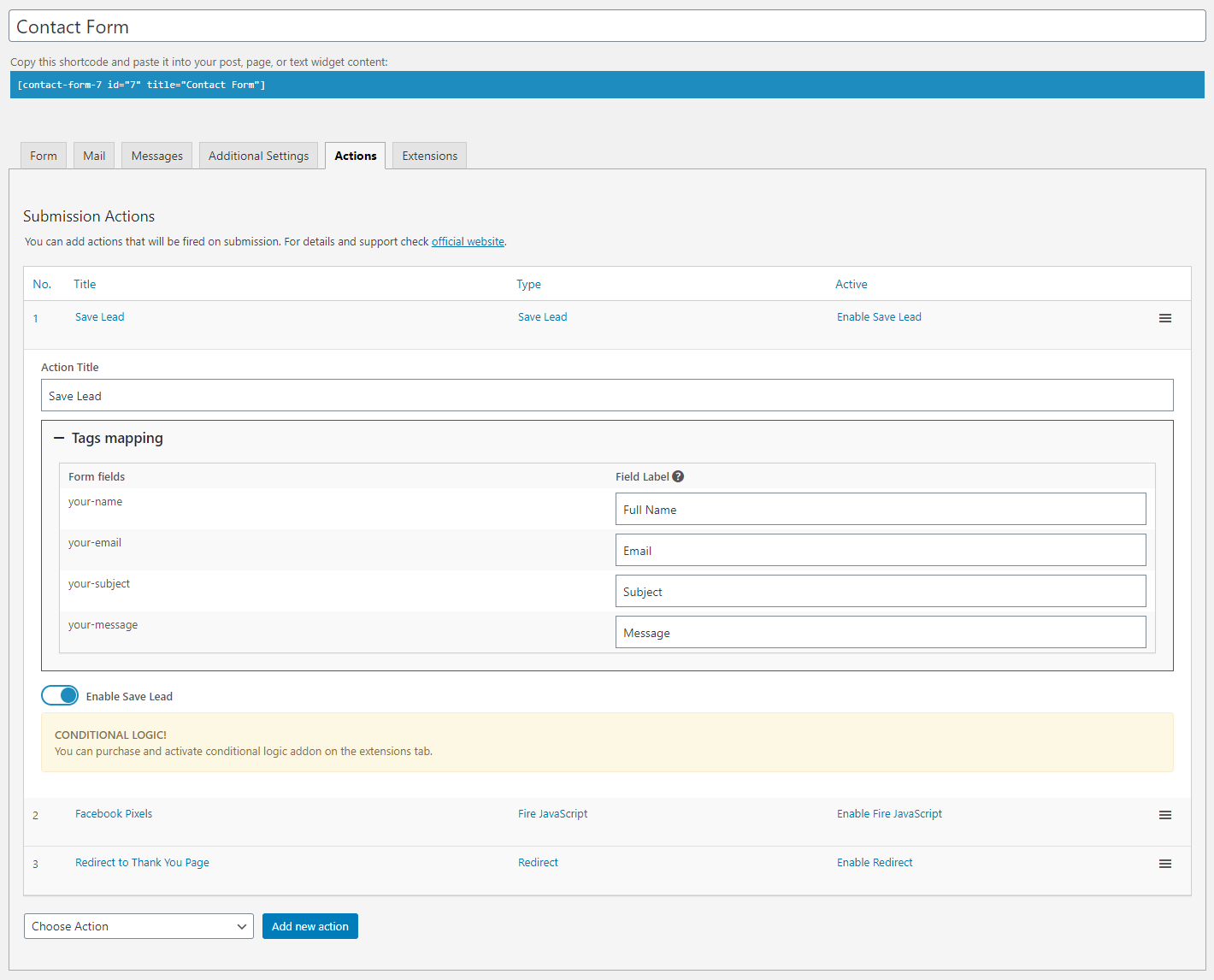This image is a detailed screenshot of a website's contact form setup interface. At the top, there is a large blank white rectangle with the heading "Contact Form" in bold. Directly beneath it, an instruction reads, "Copy the shortcode and paste it into your post, page, or text widget content." Below this directive is a blue bar containing the shortcode: 
`[contact-form-7 id="7" title="Contact form"]`.

Further down, there are six horizontal gray tabs: Form, Mail, Messages, Additional Settings, Actions, and Extensions. The "Actions" tab is currently selected, revealing a section titled "Submission Actions." In this area, users can add various actions that will trigger upon form submission. For additional details and support on configuring this feature, there is a blue hyperlink labeled "official website."